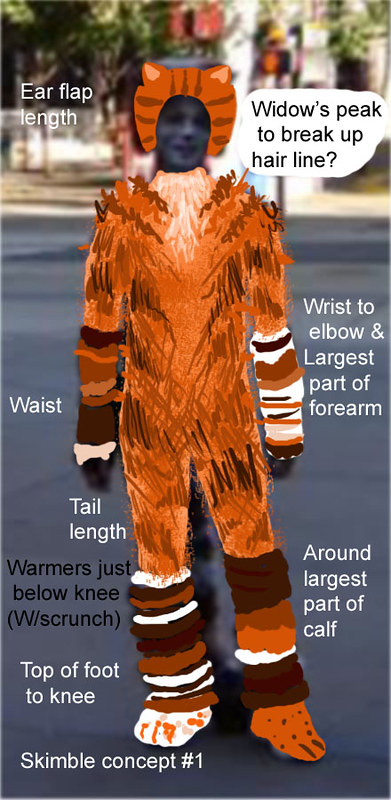The image is a combination of a color photograph and a digital drawing set in an outdoor scene featuring buildings, trees, a sidewalk, and a crosswalk sign in the background. The photograph has been overlaid with a cartoon-like illustration of a person dressed as a tiger, complete with tiger ears and a furry body, rendered in orange, brown, black, and white colors. Various measurements are labeled across the image, including "ear flap length," "widow's peak to break up hairline," "wrist to elbow and largest part of forearm," "waist," "tail length," "warmers just below the knee with scrunch," "top of foot to knee," and "around largest part of calf." Additionally, the text "Skimble Concept Number One" suggests it's a design concept for a tiger costume.